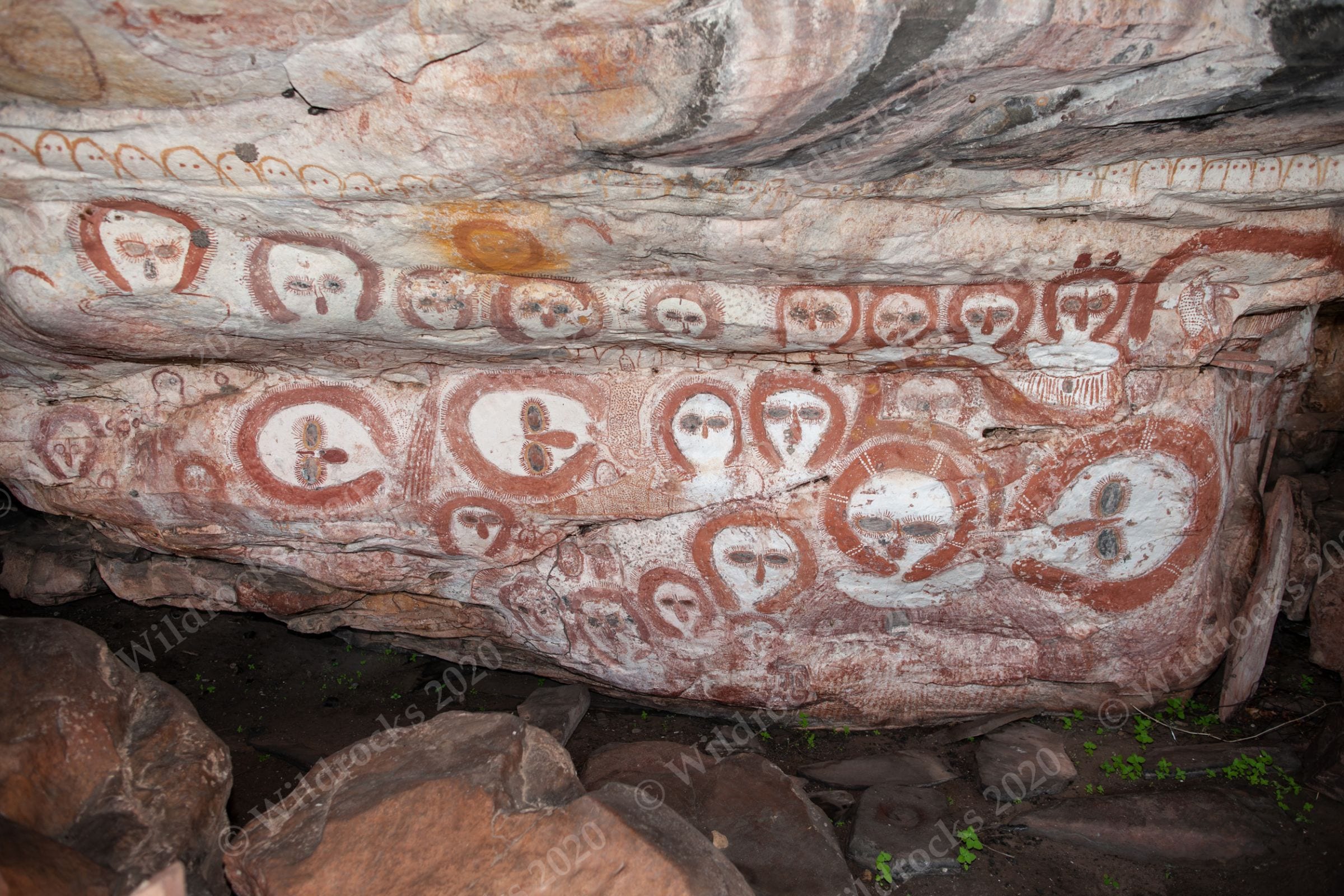The photograph depicts a close-up of a rock formation, which, at first glance, resembles an old, deteriorated mattress laying on some rocks. Upon closer inspection, it's clear that the "mattress" is actually a uniquely weathered rock surface. This rock face is intricately adorned with what appears to be historic cave paintings. Numerous white-painted heads with dark, piercing oval eyes and red or rust-colored outlines populate the formation. There are over 20 such stylized faces, giving an eerie and enigmatic appearance, reminiscent of skulls or alien-like entities. 

The background features both dark brown and lighter brown rocks, positioning the painted lighter-colored rock prominently in the composition. The rock surface is marked with white, transparent text indicating a copyright watermark that reads "Wild Rocks 2020," suggesting that it might be part of a documentation project cataloging geological and archaeological sites. The entire scene is set against a textured, compressed rock backdrop, possibly within a cave, evoking a sense of historical and artistic intrigue.